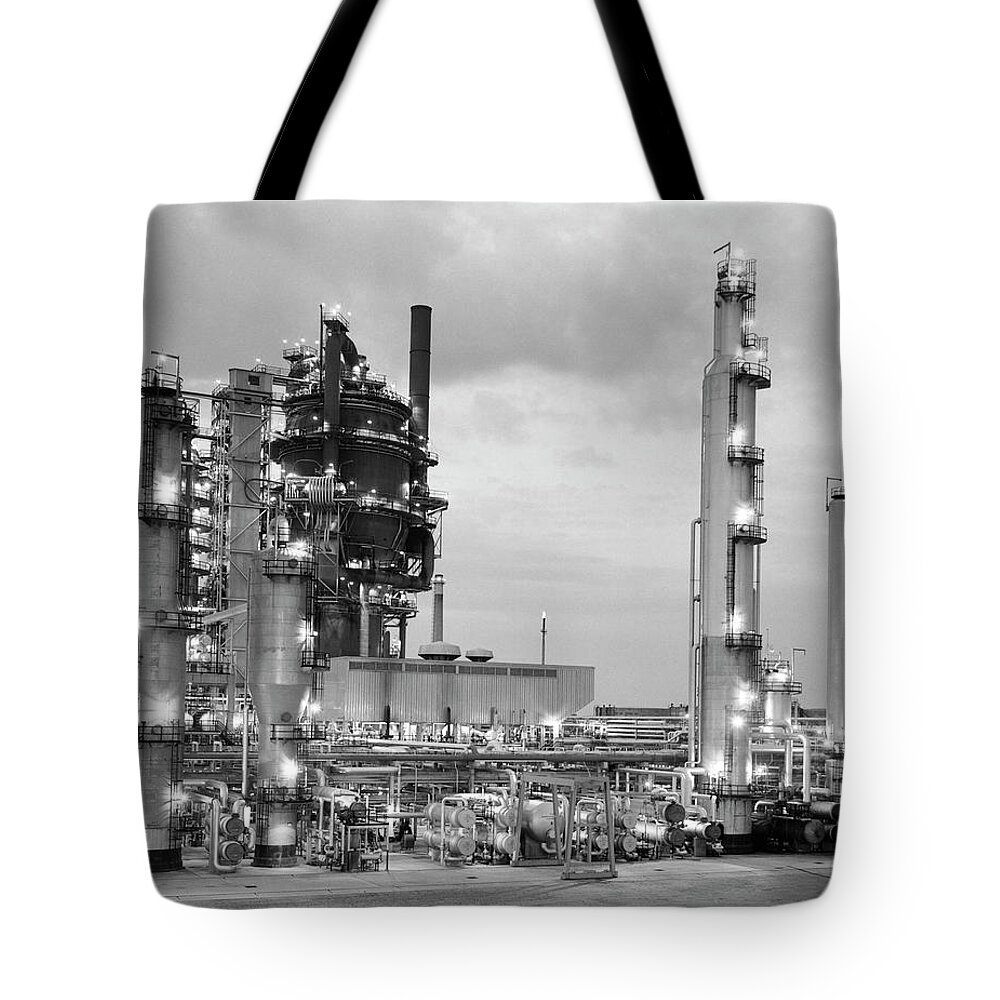This image shows a canvas tote bag with black handles in a strapped style. The bag features a detailed black-and-white image that seems to depict an industrial setting, which could be a power plant, an oil rig, or a factory. Prominent in the image are tall towers and cylindrical structures with various pipes running across the scene. A tall tower with a semi-circular platform and ladders is noticeable at the front, along with multiple staircases and lights scattered throughout the complex. Storage containers and machinery occupy the foreground, and the background shows the sky and clouds, all rendered in grayscale.